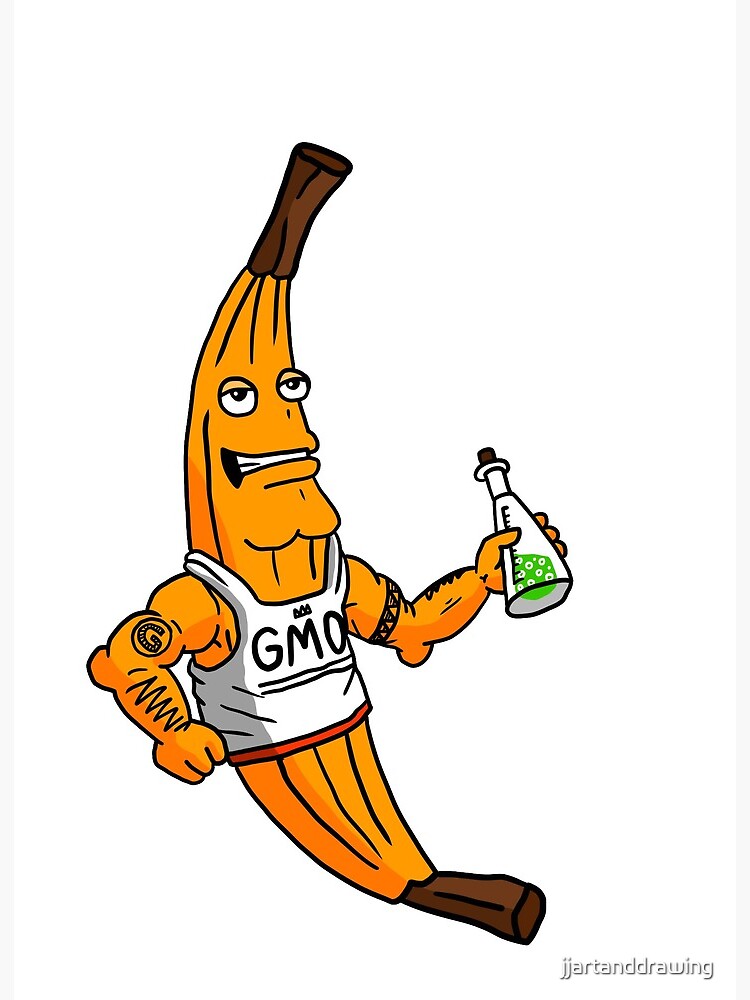This is a detailed cartoon illustration of a muscular, anthropomorphic banana wearing a white tank top with a red stripe at the bottom, emblazoned with the initials "GMO," where the "M" is topped with a small crown. The banana has a chiseled, cleft chin and a smug grin, revealing its teeth as it gazes upwards. Its skin is a dark yellow, almost golden color, with traditional brown stems at both the top and bottom. The banana has no nose or legs but boasts well-defined, muscular arms. On its right upper arm, seen on the left side of the image, it sports a tattoo of a "G." On the left arm, the banana grips a beaker sealed with a cork, containing a bubbling green liquid. The background is completely white, with semi-transparent text reading "JJADX" hovering above the banana's head, casting a shadow. The design emphasizes the surreal and humorous juxtaposition of a fruit embodying traits typically associated with superhero strength and genetic modification themes.